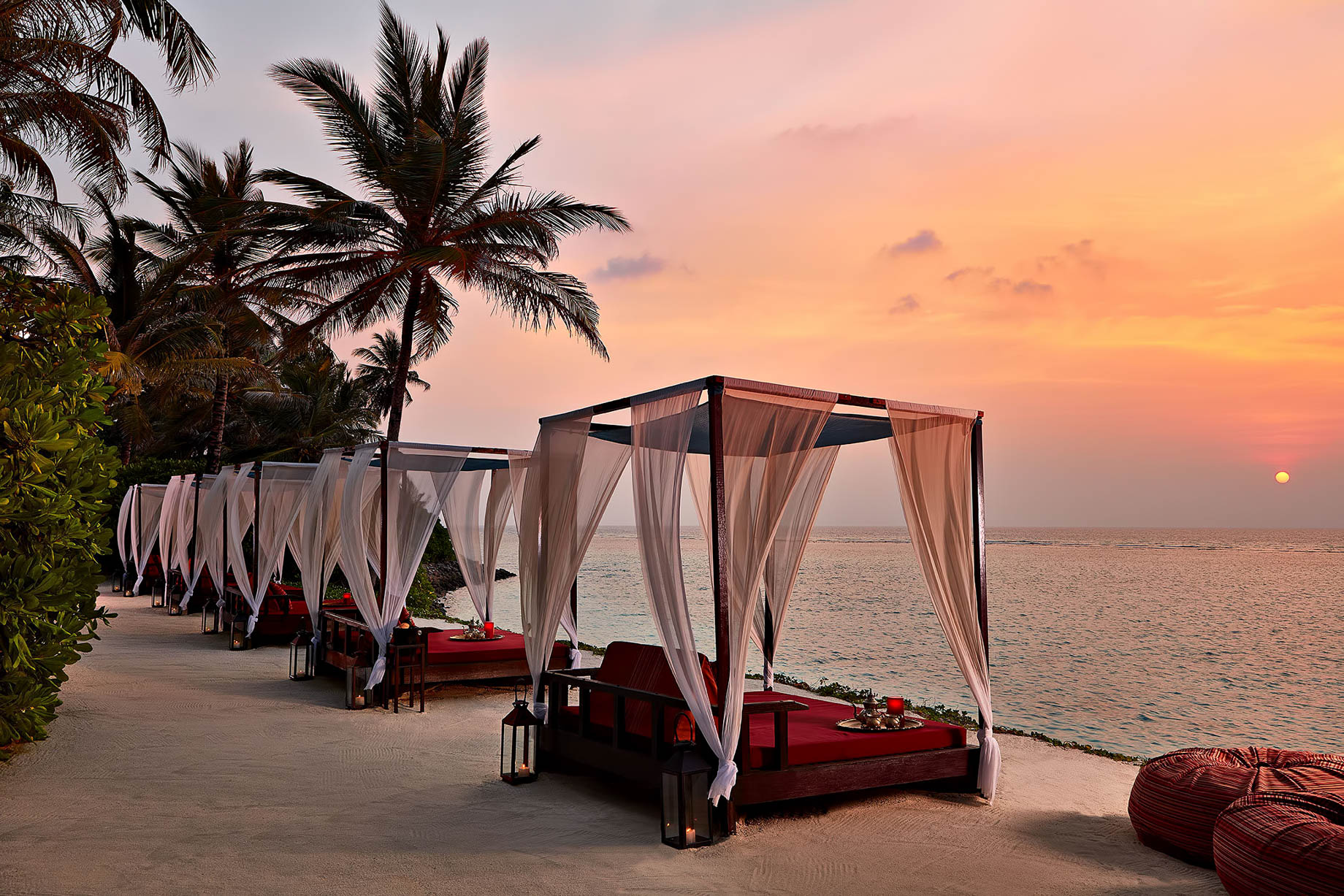This photograph captures a serene tropical coastal setting during what appears to be sunset. In the foreground, the beach is meticulously maintained, with flat, cream-colored sand that could potentially be artificial, overlaying a cement base. Lining the shoreline are eight beds, each adorned with red bed sheets and surrounded by erect structures designed to hold curtains, offering an element of privacy or shade. These beds are positioned to face the tranquil ocean, directly in front of them. The backdrop showcases lush greenery, including palm trees and a green bush. The sky displays a beautiful gradient, with a vibrant mix of gray, red, yellow, and blue hues, indicating the sun is setting near the ocean's horizon, casting an orange-yellowish glow across the scene.